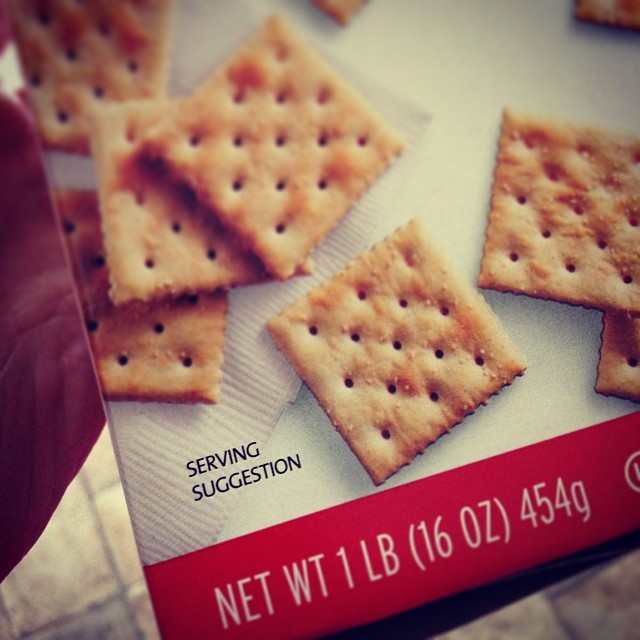The square image captures the lower left corner of a box of square, salted crackers. The front of the box prominently displays tan-colored crackers adorned with small salt crystals, set against a pristine white background that also features a white napkin. The bottom portion of the box is marked by a bold red bar extending horizontally across, which contains white text. Above this red bar, black lettering reads "Serving Suggestion" beside one of the crackers. The white text within the red border indicates the net weight as "1 lb 16 oz (454 g)." A partially visible hand, showing mainly the palm and base of the fingers of a Caucasian person, is seen holding the back of the box. The box itself is angled at approximately 30 degrees from the upper left corner to just left of the bottom center.